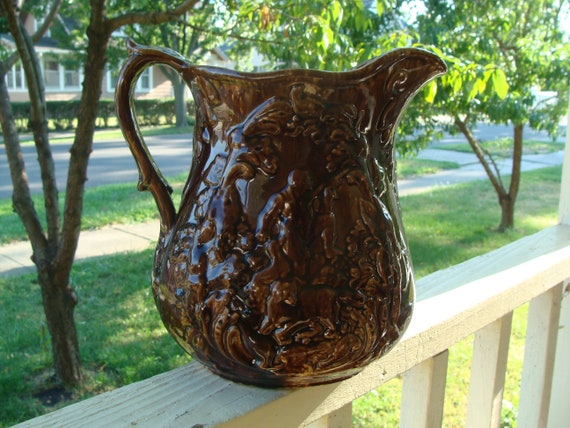This photograph captures an ornate, dark brown pitcher with a glossy, possibly slightly translucent finish, sitting prominently on an unfinished wooden railing that resembles a deck or porch railing. The pitcher features a curved top and a distinctively elaborate handle shaped like half of a heart, reminiscent of a tree branch with small nubs. The design on the pitcher is intricate and shiny, with a figure that appears to be a man engraved on its front, though the details are challenging to discern. In the background, the scene extends into a verdant neighborhood with green trees, a sidewalk, and a well-manicured lawn leading to other houses.